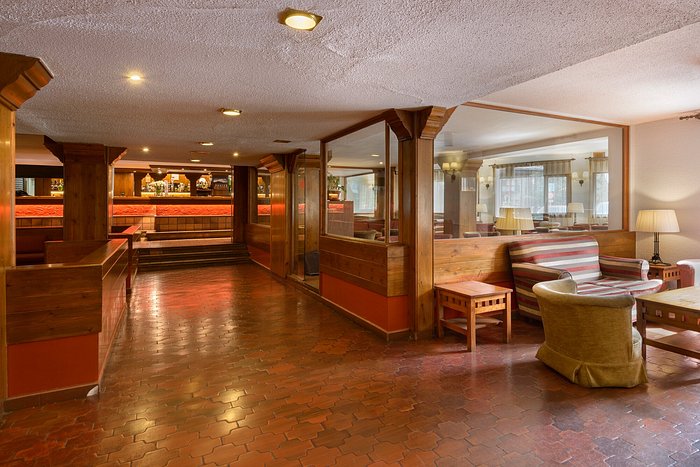This detailed and combined description captures the essence of the image: 

The photograph depicts an interior space, likely the lobby of a hotel or resort. The room features a small conversation area to the right, furnished with overstuffed tan and brown chairs and wooden end tables. A striped red, white, and brown chair is also present. The color scheme predominantly includes cream, tan, brown, and tangerine hues. The space is characterized by decor reminiscent of the late 1900s.

There is a tall lamp with a white lampshade on a table, positioned near a glassed-in area that appears to house a more private space, possibly soundproof with seats inside. The top half of the room consists of glass panels, while the bottom half is two-tone wood, combining beige with a salmon or tangerine color. The floor is covered in tangerine or clay-colored tiles arranged in a geometric pattern, resembling plus signs rather than traditional rectangular shapes.

In the background, a wooden wall features ceiling-mounted lighting and some form of imagery or artwork, which may actually be a view into another room. A tangerine-colored stripe runs across the midpoint of this wall. To the left of the image stands a large pillar extending from waist height to the ceiling, supported by a wooden half-wall that sections off another area. Overall, the ceiling is white with lighting fixtures guiding the way to what seems to be a dining area, possibly a bar or buffet. A vase with flowers adds a touch of elegance to the setting.